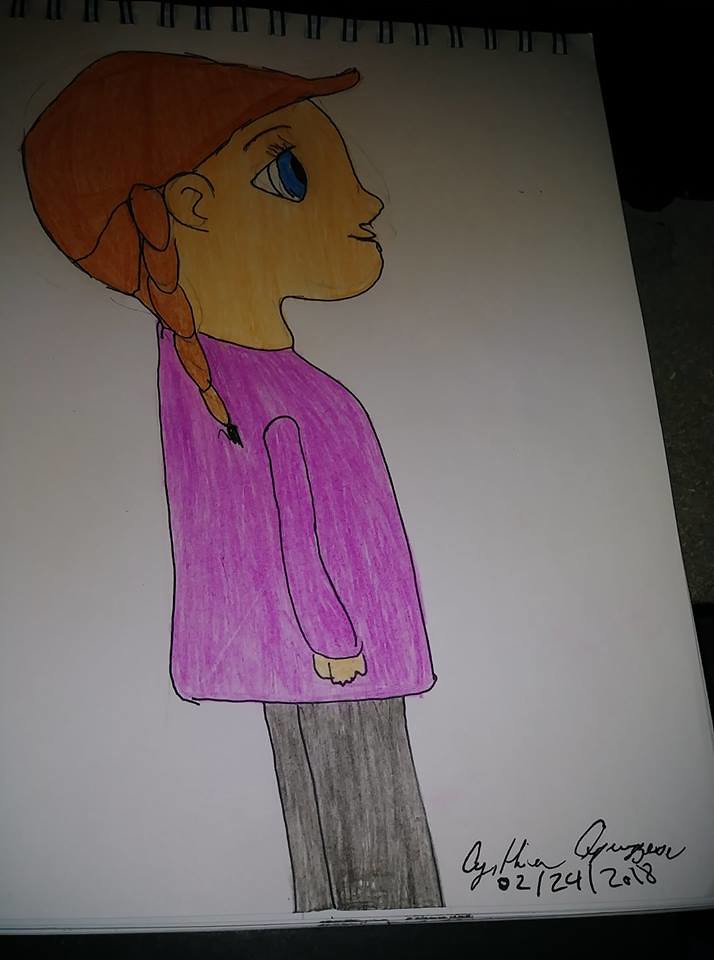This is a photograph of a vertically positioned spiral-bound sketch pad against a black background. The sketch pad features a hand-drawn, colored image of a young girl. The girl has large blue eyes, peach-colored skin, and long orangish-red hair styled in a braid or ponytail that hangs over her shoulder, ending in a black tip. She is depicted in a simple 2D style, facing towards the right side of the image. She wears a red baseball cap, a purple-pink long-sleeve shirt, and black or gray pants. The artwork, likely colored in with pencils or crayons, includes a signature at the bottom right that reads "Cynthia Aguirre," accompanied by the date "02-24-2018."